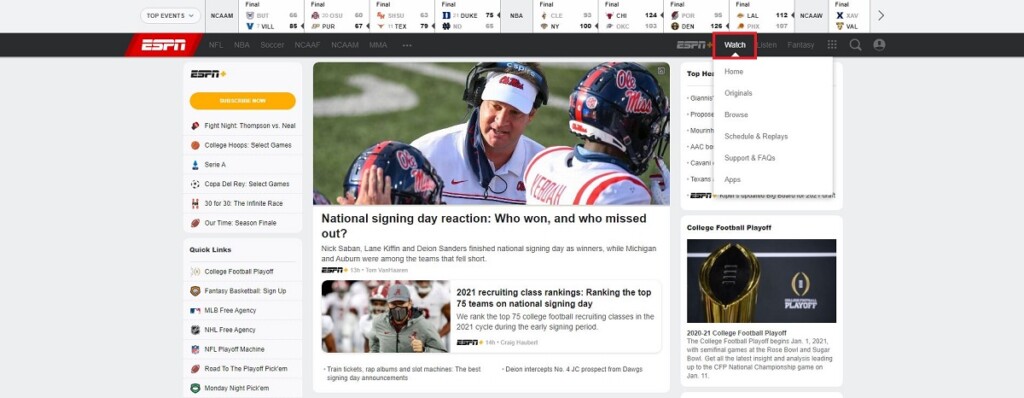Displayed on the screen is a screenshot of the ESPN website, highlighting several prominent news stories and navigational features. The central portion of the page, occupying roughly 60-70% of the width, is dedicated to the latest headlines. The leading story features an image of football players from Ole Miss, with their team name visible on their uniforms. Positioned in the center of this image, and serving as the focal point, is presumably the team's coach or kicking coach. The accompanying headline reads "National Signing Day Reaction: Who Won and Who Missed Out," indicating coverage on football signings.

Beneath this primary story is a secondary news article accompanied by a slightly smaller thumbnail. This article focuses on team rankings with the headline "2021 Recruiting Class Rankings, ranking the top 75 teams on National Signing Day."

At the top of the ESPN webpage, there's a section displaying live scores from various ongoing sports events. The scores primarily feature NCAA men's basketball games, with points ranging in the mid-60s to 70s. Additionally, scores for other games, like those involving the Chicago Bulls, are also visible.

To the left side of the main content, the website has a navigation menu providing quick links to various sections such as the college football playoffs, fantasy basketball sign-up, MLB free agency, and more.